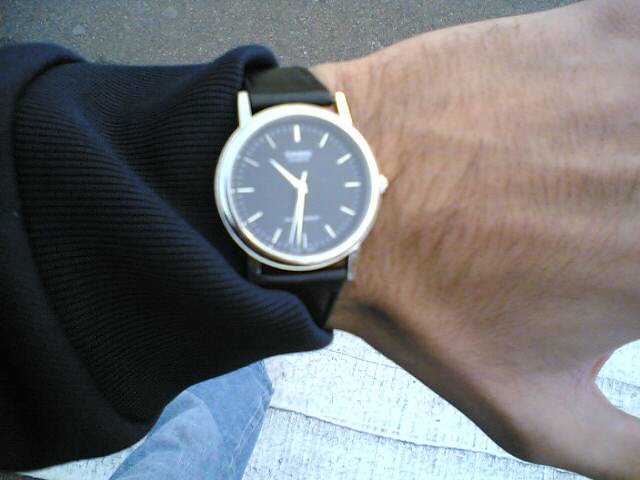This image captures the perspective from a camera attached to a man's head, offering a detailed view of his wristwatch from his point of view. His arm stretches horizontally across the center of the frame, with the focus being a stylish watch placed prominently in the middle. The watch features a gold rim and hands on a black face, which is adorned only with hash marks instead of numbers. The band appears to be black. 

The man is wearing a dark top—described variably as a sweater or sweatshirt—with the cuff visible on the left side of the image, and the hand extending to the right. Only part of the thumb and the back of the hand up to the knuckles are visible, with fingers extending out of view.

In the background, one can see one of the man's legs, clad in blue jeans, and the surface he’s walking on, which appears to be pavement or cement. The ground displays a mix of pavement and possibly some gravel, creating a textured backdrop that contrasts with the man’s attire.

Additionally, the hands of the watch indicate a time anywhere between 10:00 to 11:00 for the hour hand and 6:00 to 7:00 for the minute hand. This comprehensive look not only details the watch itself but also the surrounding elements, contributing to a well-rounded and vivid depiction of the scene.